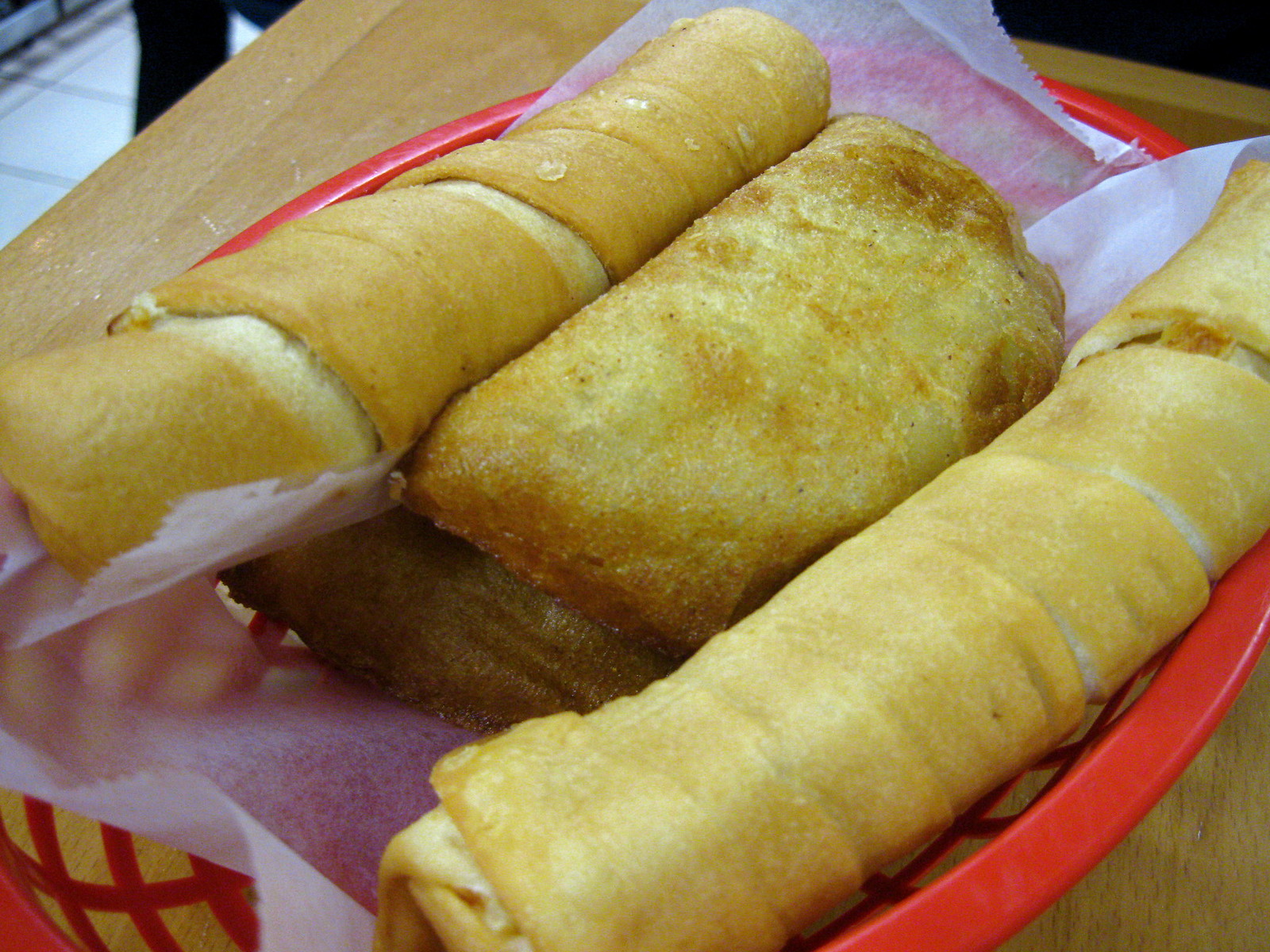This indoor color photograph is a close-up image of a basket of food placed on a wooden table, viewed from a slightly angled perspective. The focal point is a red plastic oval basket, set upon an opaque white wax paper lining inside. The basket holds three golden brown baked items, arranged carefully within. To the upper left and lower right are two cylinder-shaped rolled pasta or bread pastries. Positioned centrally is a broader, rectangular potato cake adorned with seasoning, giving it a textured appearance. Partially visible at the bottom of the frame is what seems to be a pickle. The table's light brown wooden texture is discernible in the background, particularly in the upper left and lower right corners, while a hint of a white tiled floor appears in the upper left. The food items display a uniform golden brown color, accentuated by baking, with subtle variations in their yellow golden hues. The overall scene is devoid of any text or printed material, focusing solely on the appealing arrangement of the baked goods.